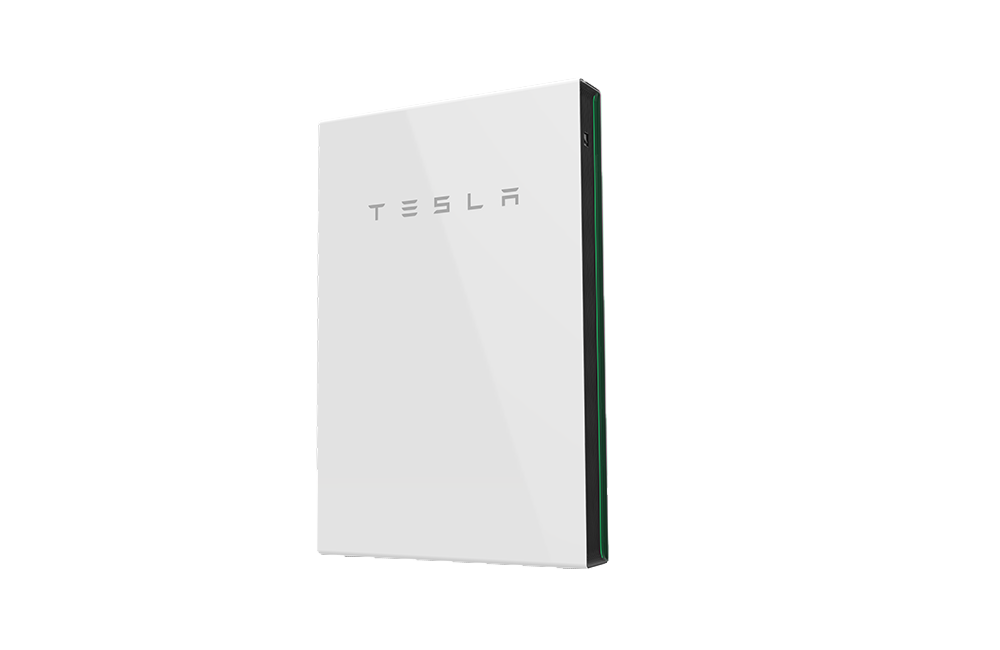The image features a sleek, vertical graphic design resembling a high-tech desktop or a sophisticated video game console. Its form factor is slender and elongated, evoking the appearance of a standing book. Prominently displayed on the side of the device is the name "Tesla," written in dark gray against a white background, identifying it as a product from the renowned car company.

The front of the device is black and features a vertical green line that runs from top to bottom, adding a touch of modern flair. This vertical line is positioned towards the right side of the device. The overall background of the image is pristine white, emphasizing the device's design.

Additionally, a distinct shadow is visible to the side, with a dark gray hue on the left and a lighter gray on the right, enhancing the three-dimensional feel of the device in the image. The Tesla branding is prominently centered at the top of the device, reinforcing its identity.